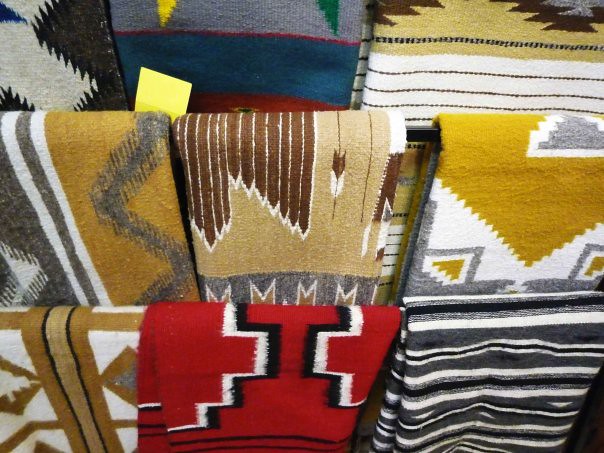The image depicts nine woven blankets or shawls, each showcasing distinct geometric designs and a variety of colors, displayed on a dark brown metal rack. From left to right, the top blanket features black, white, and gray stripes in a zebra-like pattern. The next one beside it is a vibrant red, with a white and black outline forming a T-shape and steps pattern. Moving right, there is a blanket with brown and white jagged edges, followed by another with a combination of light brown and white jagged patterns.

Continuing to the right, a blanket displays dark brown arrows on a light brown background, with a grayish base and white outlined 'M' shapes. Adjacent to it is a light brown blanket with vertical V-shaped gray patterns, interspersed with white and gray lines. Another blanket showcases light gray and reddish lines, dark blue with reddish lines, and a red section with a yellow square tag in front. 

Adding to the collection is a blanket with brown stripes and white squares outlined with black lines. Lastly, there is a distinctly patterned blanket in white with brown stripes set against a light brown and brown jagged background. The overall arrangement hints at a native American influence in the designs, blending traditional motifs with modern aesthetics.